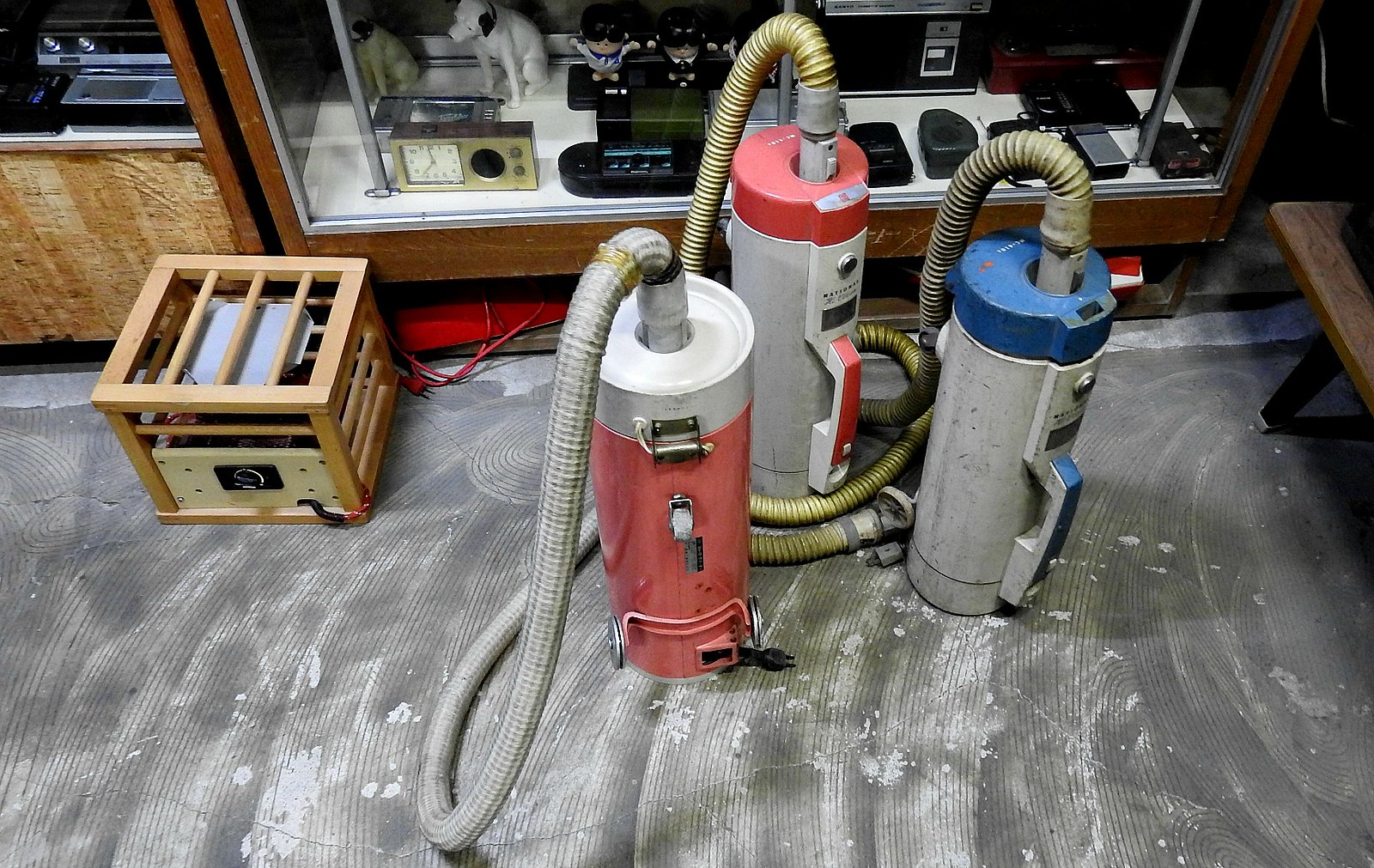This photograph appears to be taken inside a workshop or a display area showcasing old electronic equipment, possibly a museum. The floor is metallic with lots of lines across it and is very dirty, more dark grey than white, and seems to be prepared for tiling with trowel marks. In the foreground are three cylindrical vacuum cleaners, each with a flexible tubing attached. The first vacuum cleaner is red with a white top, the second is grey with a red top, and the third is grey with a blue top. These vacuum cleaners have hose cables extending from their tops. In the background, there is a display case containing vintage electronics such as an old clock radio, voice recorders, and other antique devices. On the left-hand side, there is a rectangular box with a protruding wire leading to a cabinet further back, along with various old items like an ornament of a dog and an old clock. The overall area gives an impression of a cluttered, dusty space filled with historical electronic artifacts.